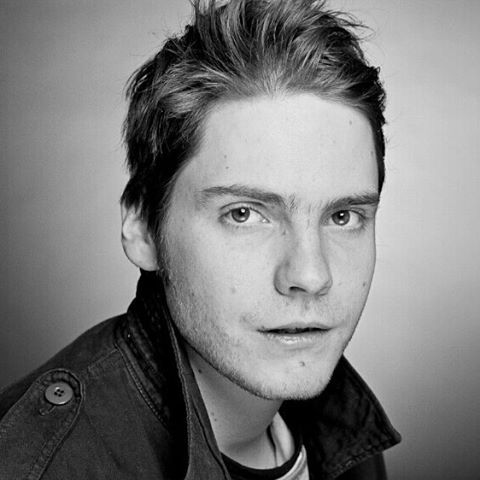The photo is a black-and-white portrait of a young man, likely in his early twenties, with light skin and dirty blonde hair styled upwards in a loose, medium length. He has a slightly stubbled face with no mustache, lending a scruffy yet clean-shaven appearance. He is wearing a dark jacket, possibly black or denim, with a distinct buttoned epaulet on the shoulder and the collar open to reveal a light or white t-shirt with a black rim at the top. The young man is gazing off to the side with a serious and earnest expression, and the background is plain and light-toned, ensuring all focus is on his contemplative pose. This image has all the hallmarks of a professional modeling headshot.